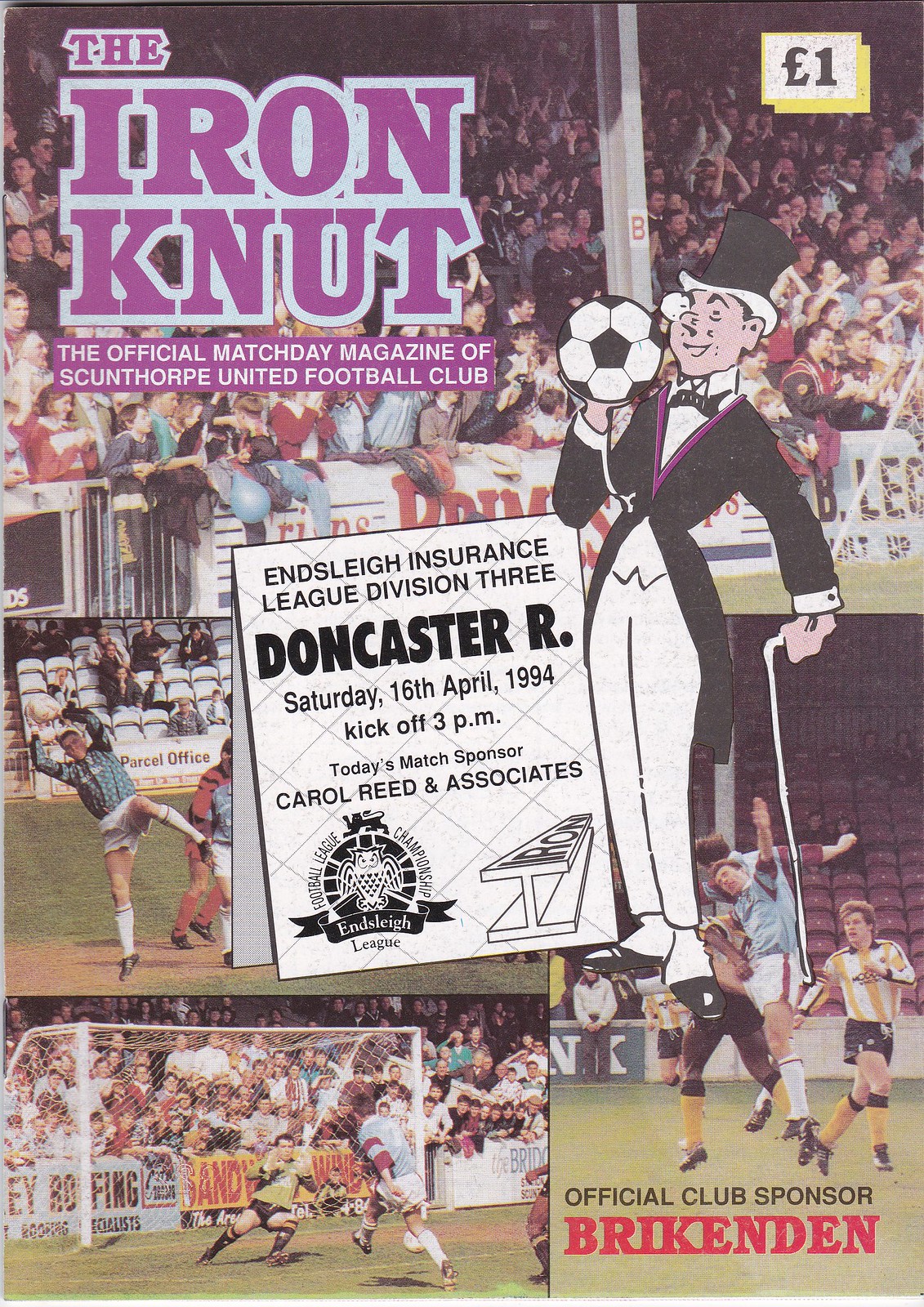The promotional material appears to be the cover of "The Iron Nut," the official match day magazine of Scunthorpe United Football Club. Dominating the top of the poster, "The Iron Nut" is prominently displayed in purple letters with a background caption that reads, "The Official Match Day Magazine of Scunthorpe United Football Club." A yellow-bordered box in the upper right corner marks the price as £1, suggesting it is British.

The background showcases various images related to soccer. At the top, a photograph depicts a crowd of fans in the stands, intently watching the game. Below this, three action shots capture the intensity of European football (soccer) matches, with players energetically engaging in the sport amidst a white goal net visible in the background.

Central to the visual is a cartoon illustration of a formally dressed man, sporting a top hat, monocle, bow tie, and a long suit jacket, holding a traditional black and white soccer ball. The left side of the cover features event specifics in a white box with black letters: "Ensley Insurance League Division III, Doncaster R., Saturday, 16th April 1994, Kickoff at 3pm. Today's Match Sponsored by Carol Reed and Associates."

In the lower right-hand corner, the magazine acknowledges its Official Club Sponsor, Brickenden, adding a final touch to the comprehensive promotional layout.